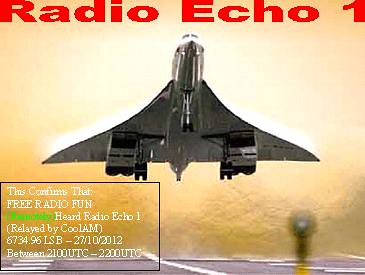The image is a realistic photograph-style card, designed for radio enthusiasts and operators. Dominating the card is an impressive shot of an airplane closely resembling a Concorde jet, captured at the moment of takeoff against a golden-yellow background. The perspective is from the runway, showing the jet angled upwards as it ascends, with its underbelly and extended wheel assembly clearly visible. The aircraft, mostly white with shaded underparts, exhibits the characteristic thin, pointed nose and backward-swept wings of the Concorde. Noteworthy, the text "Radio Echo One" is prominently displayed in red at the top. In the bottom left corner, a black outlined rectangular box contains details in white and green text. The text confirms the reception of "Radio Echo One" relayed by "Cool AM," with recorded details including the call sign LAM 6734.96, the date 27-10-2012, and the time frame between 2100 UTC and 2200 UTC. Additionally, there is a blurred image of a man located at the bottom right corner of the card.